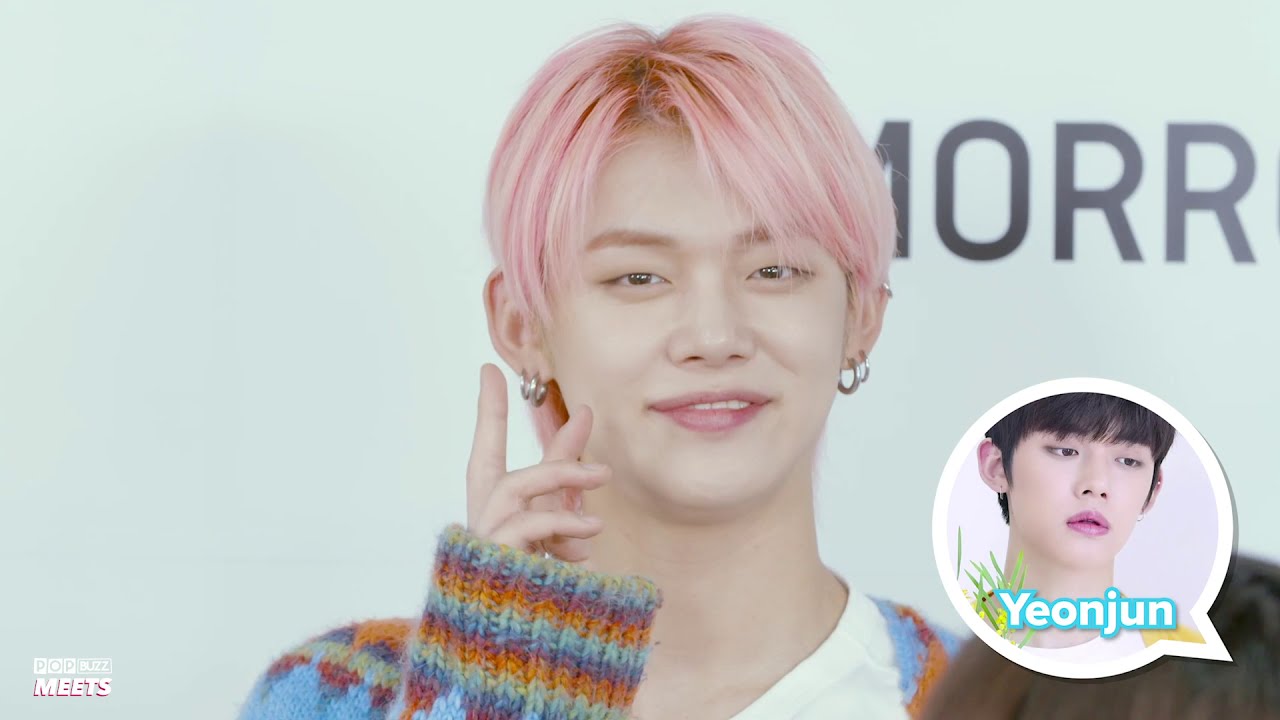The photograph features a fair-skinned, young Asian man with straight pink hair that partially covers his eyes and ears. He is adorned with multiple silver hoop earrings—two on each earlobe and one additional on the upper lobe of his right ear. His makeup includes pink lipstick or lip gloss. The man is smiling at the camera with his right hand raised in an open gesture, reminiscent of a peace or V sign. He is dressed in a blue fuzzy sweater with orange and purple stripes, layered over a white T-shirt. Behind him, a partially visible wall displays the text "M-O-R-R" in black letters, set against a light mint green backdrop. In the upper right corner of the image, a speech bubble reveals another young Asian man with dark black hair, looking downward. His name, "Yeonjun," is inscribed beside him in white text with a blue outline. The bottom left corner of the image includes the small-print words "Pop Meets." Overall, the scene exudes the polished and vibrant aesthetic typical of K-pop stars.